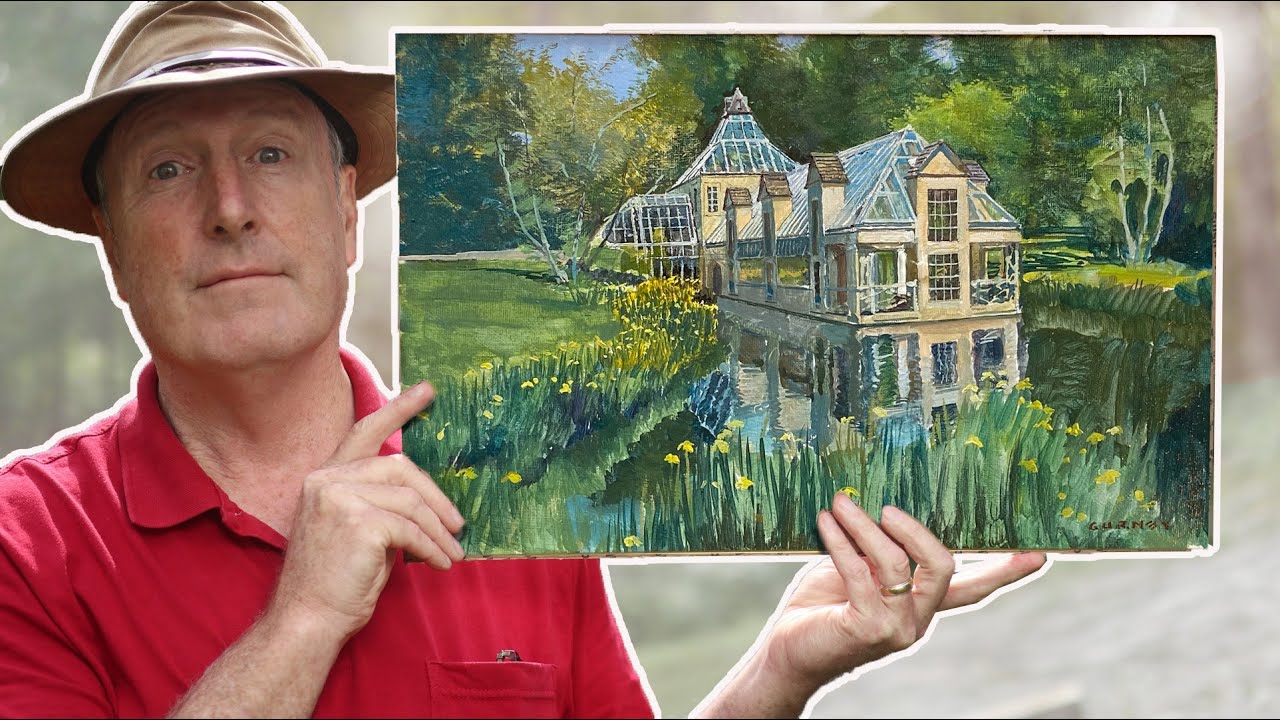In the image, a middle-aged white man, estimated to be in his 40s to early 50s, stands on the left side. He has green eyes, gray hair, and a square jaw, and is wearing a tan hat with a full, circular brim. Dressed in a red collared polo shirt with three buttons down the front and a pocket on his right chest, he holds a painting with both hands.

The painting portrays a tranquil lakeside scene featuring an architectural structure, which seems to be a boathouse or a glass-roofed lake house positioned in the center. The house is designed with a significant amount of glass, including a rectangular glass roof and additional glass elements on the sides, as well as a triangular section at the back. The serene water surrounding the house reflects the lush greenery and yellow flowers that adorn the scene. 

Behind the house, a gentle green hill slopes down to meet the structure, while the background features trees and a possible dirt road in front. The calm lake or pond cradles two boats moored at the boathouse, complementing the peaceful atmosphere depicted in the painting.